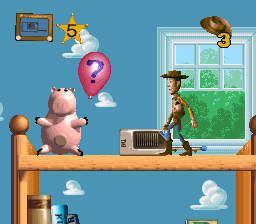In this vibrant image from a mobile game centered around characters from the movie Toy Story, we find the iconic cowboy doll Woody and the piggy bank toy Hamm perched atop a wooden bookcase. Below them, a row of colorful books occupies a lower shelf. Sharing their space on top of the bookcase is a silver and black walkie-talkie.

Floating above these beloved characters, a series of whimsical objects add an element of playfulness to the scene: a gold star with a number five on it, a balloon adorned with a question mark, an Etch-A-Sketch, and a cowboy hat featuring a number three. The background showcases a cheerful blue wallpaper with a cloud motif, enhancing the lively, imaginative atmosphere. Behind Woody, an open window reveals a scenic view of the blue sky and lush greenery, adding depth and context to the setting.